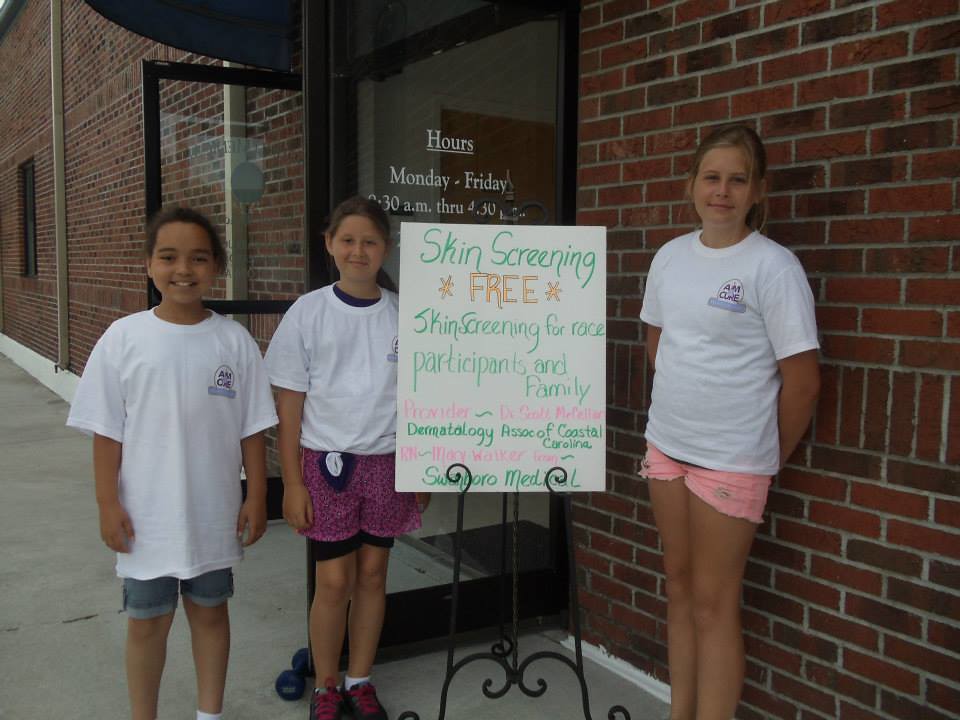The image captures three young girls, estimated to be around 8 to 13 years old, standing outside a brick building with open glass doors framed in black trim. A small purple dumbbell holds the right door open. The girls, dressed in white t-shirts with the branding "AM Cure" in the top right corner and wearing shorts, all smile warmly at the camera. They flank a black metal display stand with a white sign that features prominently written green text reading "SKIN SCREENING" at the top. Below this, in yellow, the sign announces "FREE" skin screenings for race participants and their families. Additional information in pink and green mentions a provider's name, the "Dermatology Association of Coastal Carolina," and "Swanboro Medical" at the bottom of the sign. The scene is set on a grey sidewalk outside the entrance, adding a cohesive backdrop to the girls’ cheerful demeanor and the important community health message displayed.